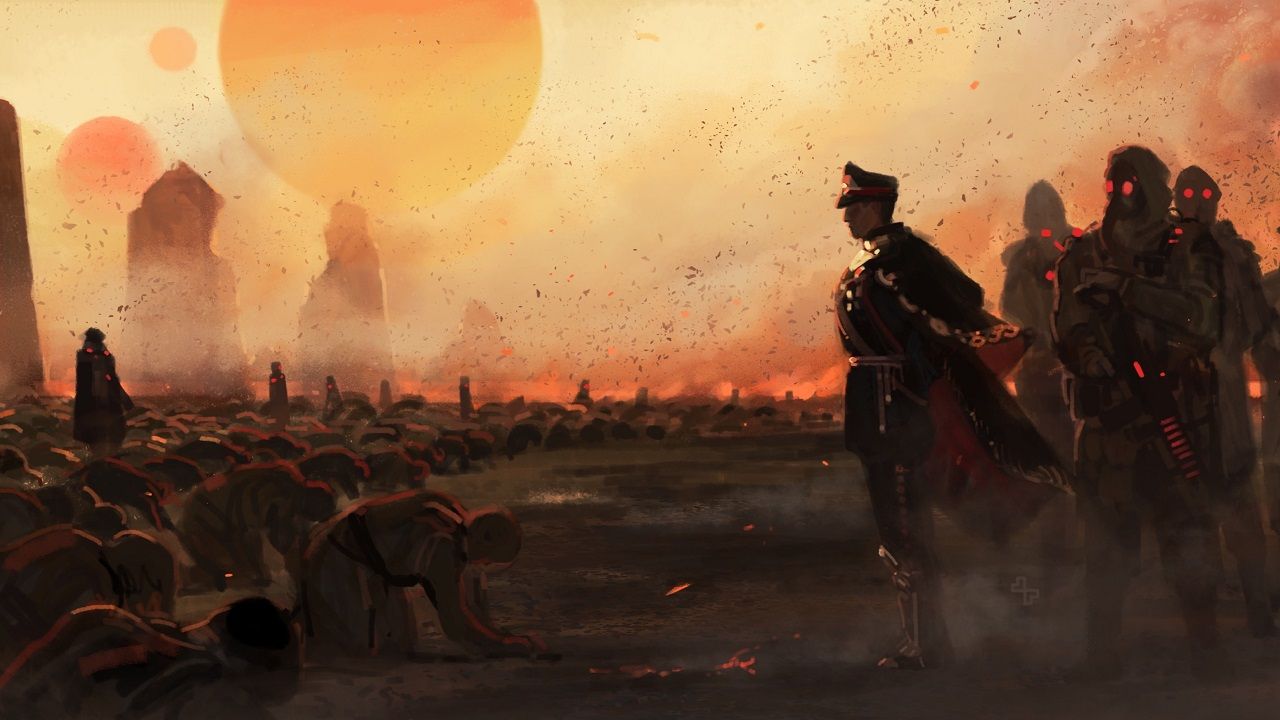This landscape-format, color illustration, imbued with an orangish tint, appears computer-generated and was likely created using tablet or computer software. It depicts a dramatic sci-fi scene characterized by a clear structural imbalance. On the right side, a commanding figure dressed in a stylized military uniform, complete with cape and boots, stands majestically against a stormy, windswept background. His profile view shows him looking left towards a crowd of defeated individuals bowing down to him in subjugation. These individuals, clothed in simple, tattered robes, represent the vanquished poor.

Behind the authoritative figure are three soldiers clad in toxic waste suits, each with glowing goggles reflecting the fiery, smoky sunset that dominates the otherworldly, toxic landscape. The background reveals a tumultuous sky scattered with multiple celestial bodies and rugged mountains, adding to the surreal, dystopian atmosphere. Overall, the image is dense with shadows and contrasts, highlighting the defeated, toxic environment in which this unsettling scene unfolds.